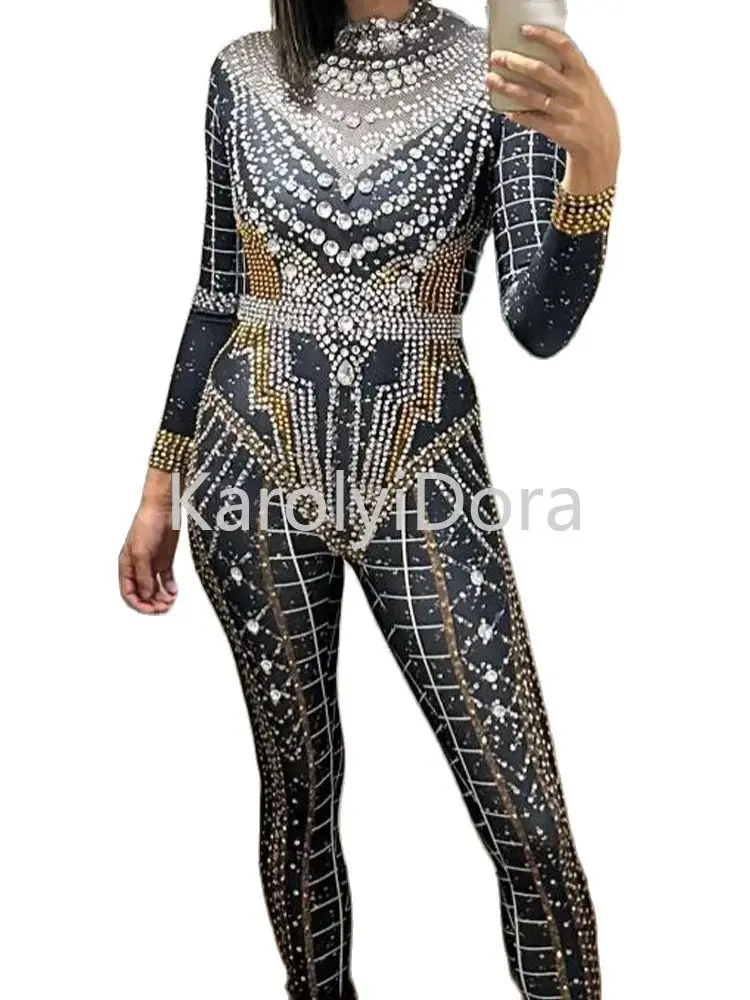In the image, a woman is taking a full-body selfie to showcase an extravagant, long-sleeved, and long-legged black bodysuit adorned with a plethora of jewels and embellishments. The bodysuit features intricate patterns formed by rhinestones in varying shades of silver, gold, and bronze, with specific orange and yellow lightning bolt designs that start at the ribs and run down to the crotch. These lightning bolts are outlined in white, adding a striking visual effect. The neckline of the bodysuit is particularly ornate, with jewel patterns resembling necklaces, while gold beads around the wrists mimic multiple bracelets and silver beads accentuate the elbows. Additionally, a graph-like pattern decorates the inner thighs to the edges of the visible leg area, although the feet are cut off in the image. The woman's neck and a glimpse of her hair, which appears brown or dark blonde with black undertones, are visible, but her face is not. She appears to be taking the selfie in a mirror, holding the camera in her left hand while her right hand rests at her side. The image also has a watermark with the text "Karolyi Dora," presumably the name of the designer or the user who uploaded the photo.